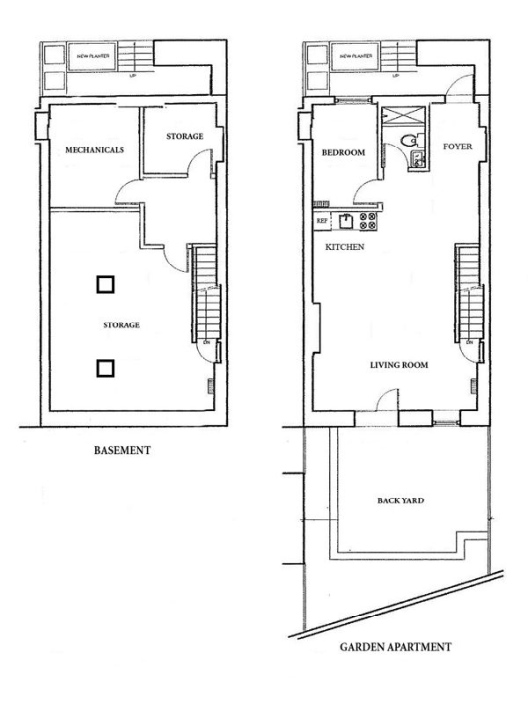This is a detailed floor plan illustrating both a basement and a garden apartment, presented in a black and white schema. The floor plan highlights the walls, doors, stairs, and certain appliances with black lines, and the labels are marked in black font. Both the basement and the garden apartment appear to share similar dimensions. 

For the basement area, it comprises a mechanical room, a storage room, and another storage area that features two central pillars, indicating structural support. 

The garden apartment on the first floor includes several distinct spaces: a bedroom, a foyer, and a living room. There is also a staircase that presumably connects to the basement level. Additionally, the garden apartment is attached to a backyard, which further extends to a garden area, offering an outdoor extension to the living space.